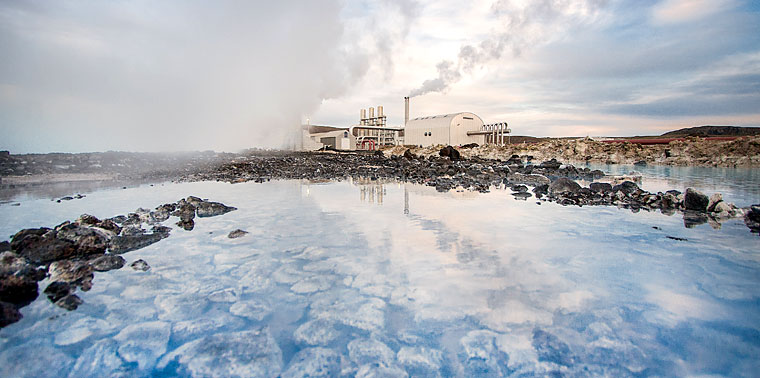This rectangular, landscape-oriented photograph captures a detailed view of a thermal electric plant. In the foreground, the clear water reveals large boulders and stones beneath its surface, with some black rocks emerging along the shores. The horizon is dominated by the plant, a large, white, warehouse-like structure with multiple pipes and smokestacks, from which smoke is visibly emanating. Additional white buildings are situated to the left of the central plant structure. Above, a sprawling sky exhibits a gradient of light blue, interspersed with pink and gray clouds. To the far left of the photograph, a sweeping wall of fog is beginning to encroach upon the scene, contrasting with the otherwise tranquil water and the imposing industrial architecture.